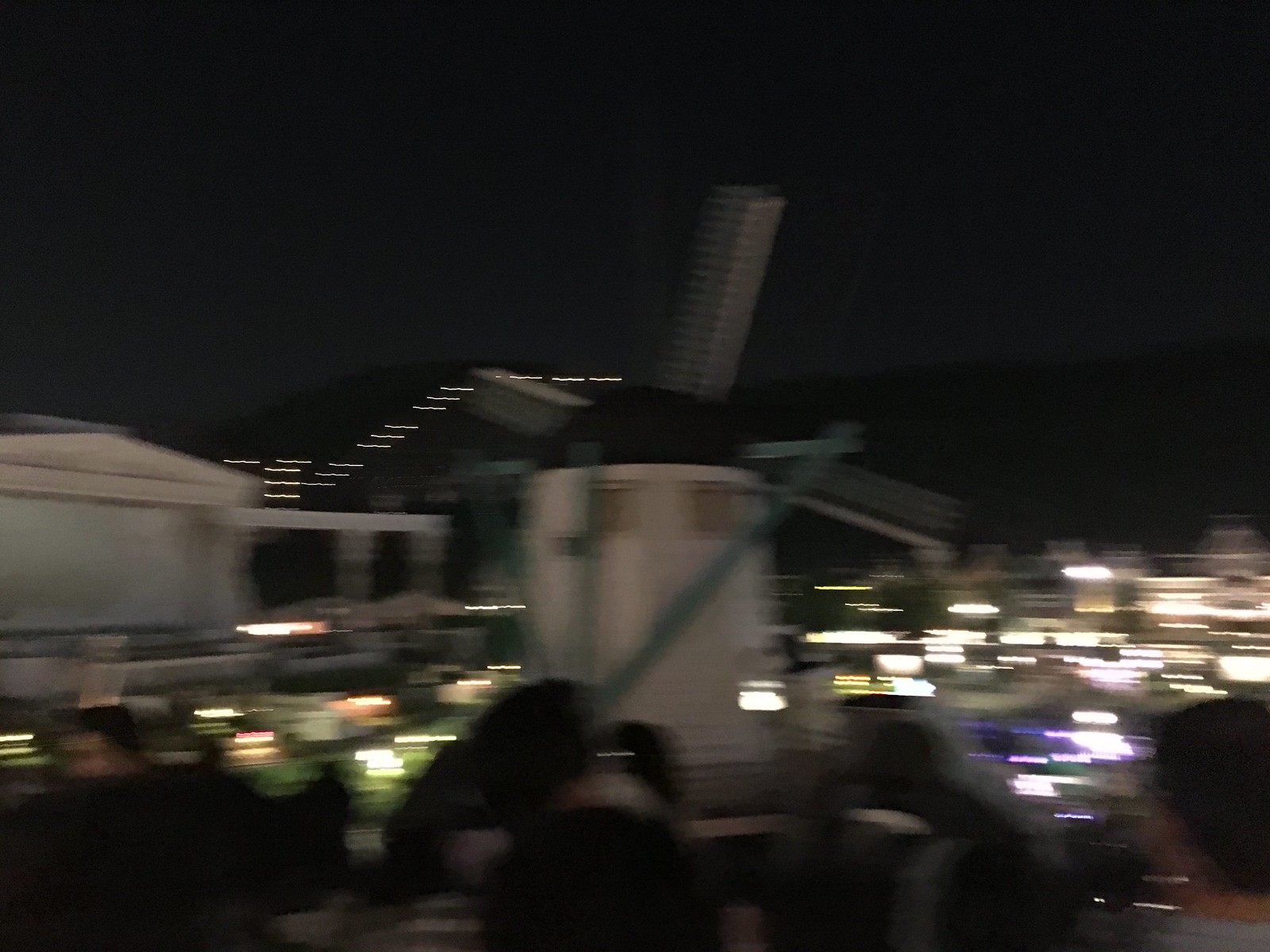In this nighttime, slightly blurry photograph, a small windmill, reminiscent of those found on mini golf courses, stands prominently in the center. The windmill features a white cylindrical base topped with a black dome. Three gray bars frame the windmill, with one extending upwards through the middle and two angling outward to the sides. The upper section of the windmill is adorned with small square windows encircling the dome, and three of the windmill's blades are visible. Behind the windmill, blurry lights create a soft, illuminated backdrop. In the foreground, several people are gathered around the base of the structure. To the left, a white building with an extended roof supported by columns is partially visible. The scene is bathed in the darkness of night, with a dark sky completing the backdrop.